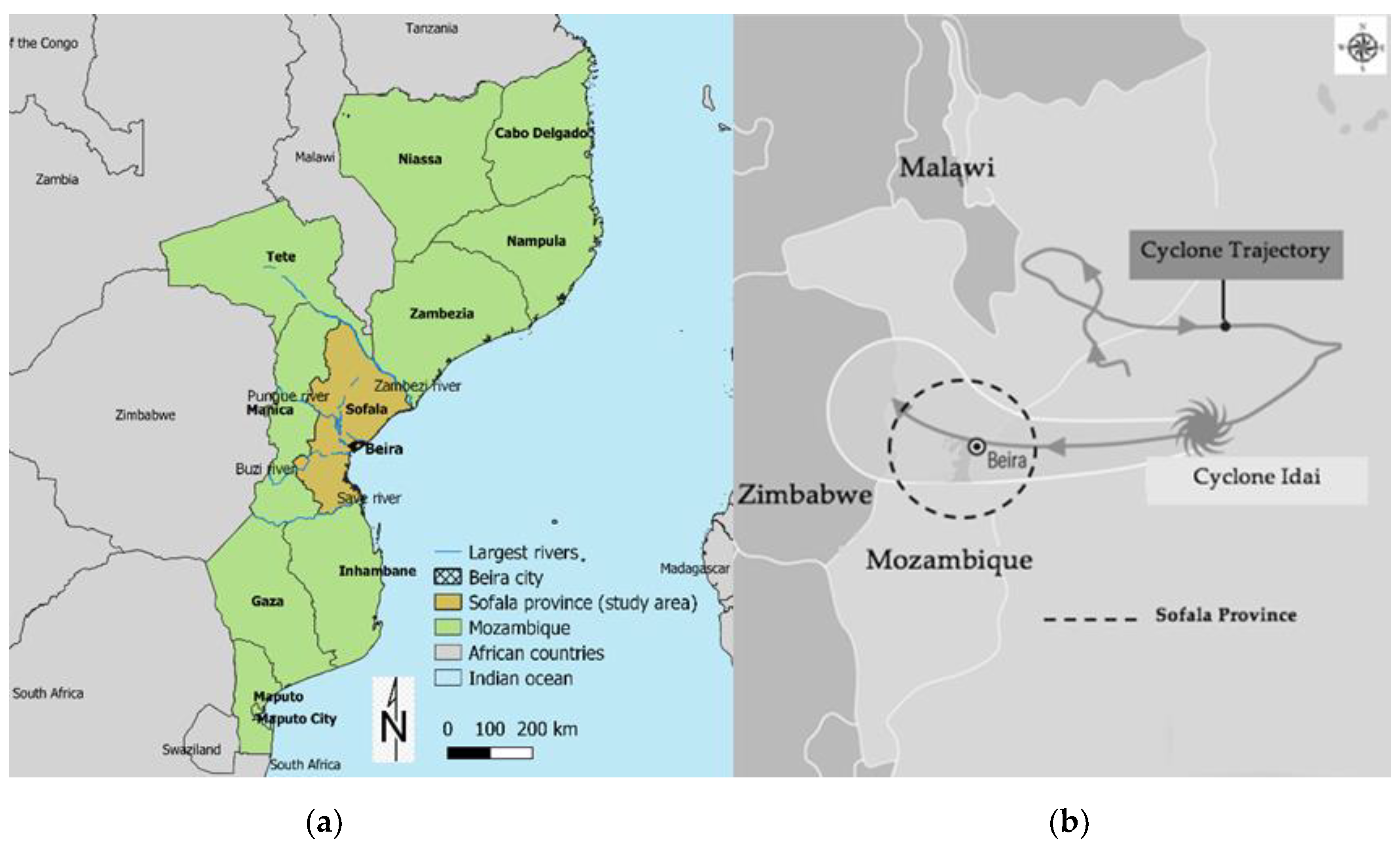The image features two maps side-by-side highlighting different aspects of the southeastern region of Africa. The first map on the left, labeled as A, depicts various countries with distinct color sections, including gray, white, and brown, indicating different areas and possibly ecological or geographical regions. Notable territories such as South Africa, Mozambique, and the Indian Ocean are labeled, along with graphics illustrating important features like largest rivers. The second map on the right, labeled as B, is an all gray map marked with black writing, light gray, and dark gray colorations, primarily focusing on Mozambique, Zimbabwe, and Malawi. This map incorporates a weather graphic that shows the projected trajectory of Cyclone Ida, with circles indicating key affected areas, such as Mozambique and Vieira. The maps together provide a detailed visual blend of geographic boundaries and meteorological data for the region just below Tanzania.